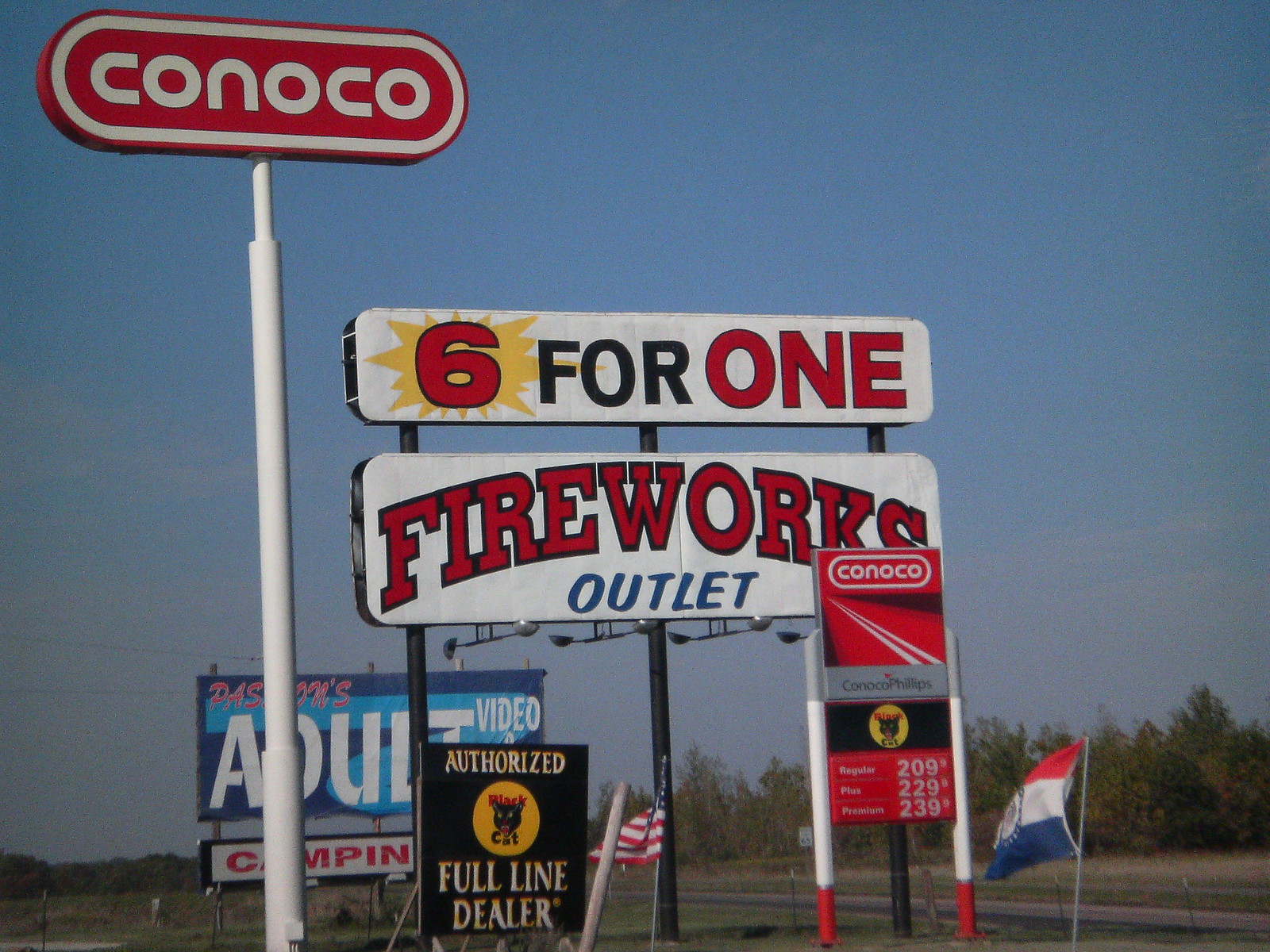This image features a Conoco gas station sign prominently displayed in the foreground. The main sign is a large red rectangle mounted on a white pole, boldly reading "Conoco" with the company's logo. Beneath this, there's a smaller rectangular price sign, also red with the Conoco logo, detailing fuel prices: Regular $2.09, Plus $2.29, and Premium $2.39. Adjacent to the gas station signage, a vibrant red, white, and blue flag flutters. Below the flag, a black sign reads "Authorized Full Line Dealer," along with an image of a black cat logo. Surrounding the area are large white and red signs advertising a "Six for One Fireworks Outlet." In the background, partially obscured, is a sign advertising adult videos, providing a contrasting backdrop to the gas station foreground.